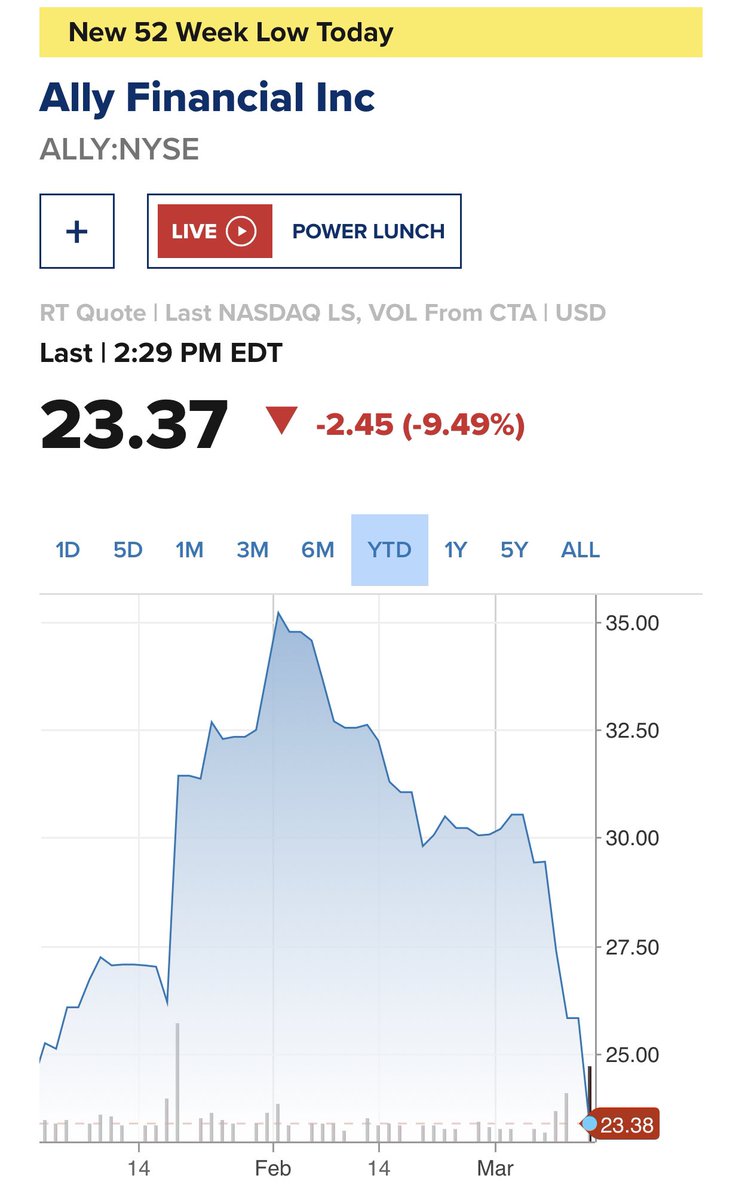The image is a detailed smartphone screenshot focusing on a financial alert. At the top, there is a yellow banner with black text indicating "New 52-week low today." Below this banner, the background turns white and prominently displays "Ally Financial, Inc." alongside the stock symbol "ALLY: NYSE." 

Beneath this information, a red rectangle with white text states "Live," implying real-time data. To its right, still on a white background, is the label "Power Lunch." Directly below, the stock price is indicated as $23.37. A red inverted triangle, accompanied by red text, shows a decrease of $2.45 and a percentage drop of 9.49%, illustrating a significant decline in stock value.

At the bottom of the screenshot, a graph visualizes the stock price trajectory. It suggests a peak near $35 but currently reveals a steep downward trend, hitting what appears to be an all-time low.